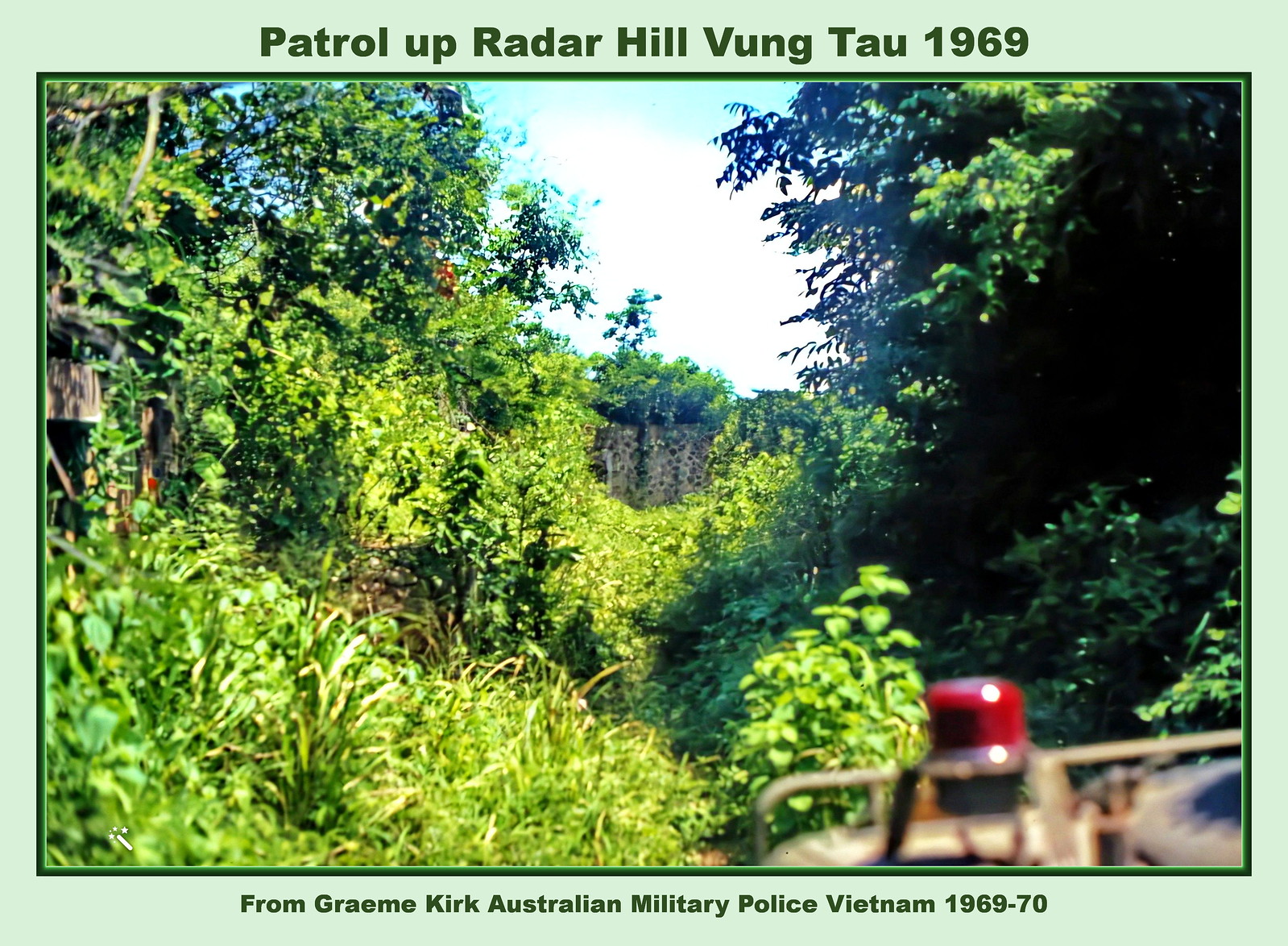This vibrant full-color photograph captures a scenic wilderness landscape on a bright, sunny day, reflecting the lushness characteristic of spring or summer. The foreground features dense clusters of trees and bushes, providing a rich tapestry of verdant greens. In the background, subtle formations suggest the presence of small cliffs, although their details are somewhat obscured. The image is marked with "Patrol up Radar Hill, Phuong Thao 1969" at the top, indicating the location and date.

In the bottom portion of the photograph, the front of a Jeep adorned with a distinctive red siren, suggestive of its use by the military police, comes into view, adding a dynamic element to the composition. An inscription at the bottom identifies the scene as being from the collection of Graham Kirk, who served with the Australian Military Police during the Vietnam War in 1969. This historical context enriches the image, blending natural beauty with a poignant slice of military history.